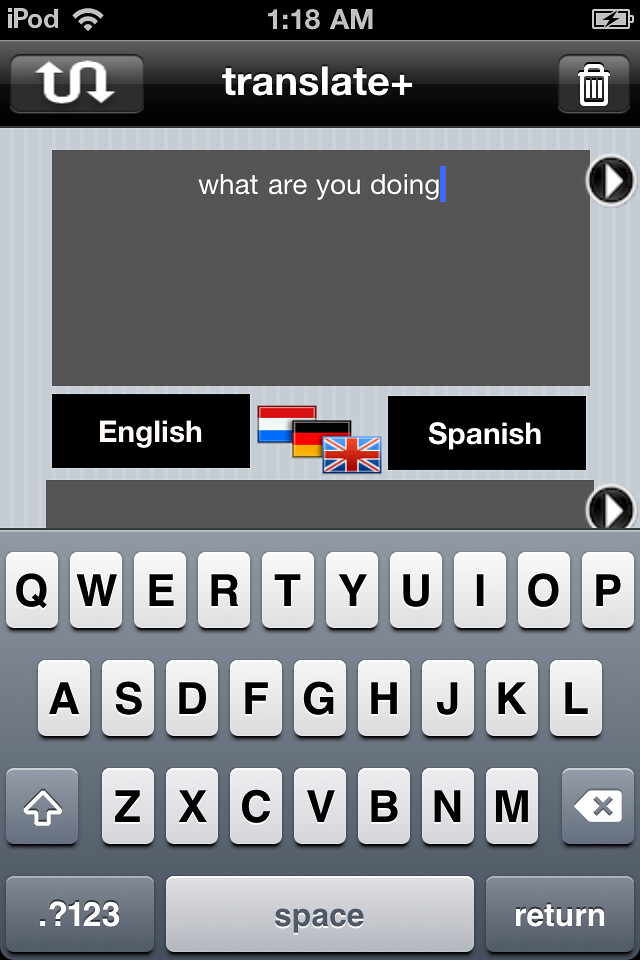The image is a detailed screenshot from an older iPod Touch, displaying the "Translate Plus" app. At the top of the screen, a thin black bar shows the status indicators: "iPod" with a full-strength Wi-Fi signal on the upper left, 1:18 AM in the center, and a fully charged battery symbol that is still charging on the upper right. Below this bar, the app interface is visible with the "Translate Plus" title at the top. Beneath the title, there is a prominent gray text box containing the text "What are you doing?" This is followed by two black selection boxes — "English" on the left and "Spanish" on the right — indicating the languages for translation.

Between the language boxes, three flag icons are displayed: the British flag for English, the German flag, and another that could be interpreted as the Netherlands or possibly the French flag due to the overlap in descriptions. This suggests that multiple language options are available in the app.

The bottom half of the screen showcases a virtual on-screen keyboard with a classic, simplistic design. The keys appear as white rectangular boxes with black lettering, and functional keys such as the space bar (in silver), backspace, shift, numbers, and return are distinguished by gray boxes with white text. The overall interface looks dated, suggesting it's more than a decade old, evidenced by the old-style 3D effects and shadows typical of early iPod and iPhone designs.